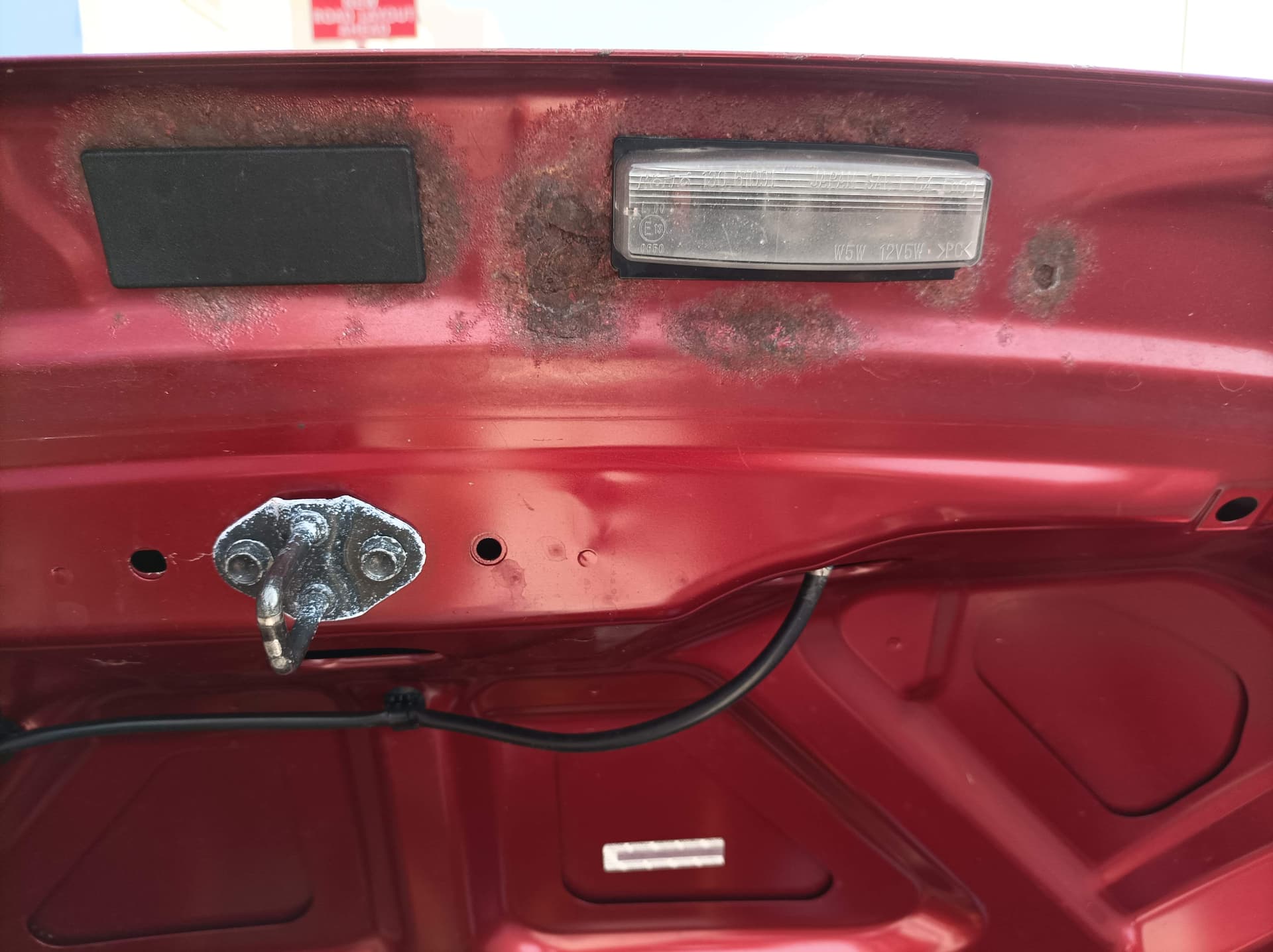The photograph features the underside of an elevated red car trunk lid, revealing several detailed components. Prominently visible is a light positioned towards the bottom right, surrounded by noticeable rust formation edging the trunk’s top and spreading throughout the metal surface. A metal clasp or latch mechanism, essential for securing the trunk, is situated near a red cord or wire threading through a hole, likely intended for the light. The image also contains a magnetic or metallic pad likely part of the locking system. Additionally, there are several holes and a black square contributing to the structure's integrity, alongside numerous rust spots and signs of wear. The scene is illuminated by daytime light, enhancing visibility of the wear and rust. The trunk’s condition indicates a need for maintenance.